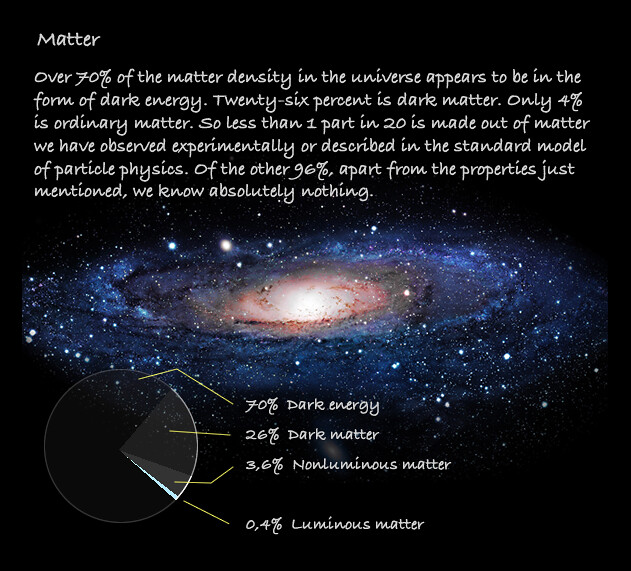This is an educational poster with a predominantly black background featuring a detailed visual and textual representation of matter in the universe. Central to the design is an image of the solar system, effectively framed by a header that reads "Matter." Above the image, a block of text, styled to resemble handwritten notes, explains that over 70% of the matter density in the universe is dark energy, 26% is dark matter, and merely 4% is ordinary matter. This text emphasizes that less than one part in 20 is composed of matter that can be observed experimentally or described by the standard model of particle physics, and expresses our lack of knowledge about the remaining 96%. Beneath the solar system image, in the bottom left corner, is a pie chart with sections indicating 70% dark energy, 26% dark matter, 3.6% non-luminous matter, and 0.4% luminous matter. The poster's composition and informative content suggest it is designed for educational purposes, likely to be displayed in a classroom setting.